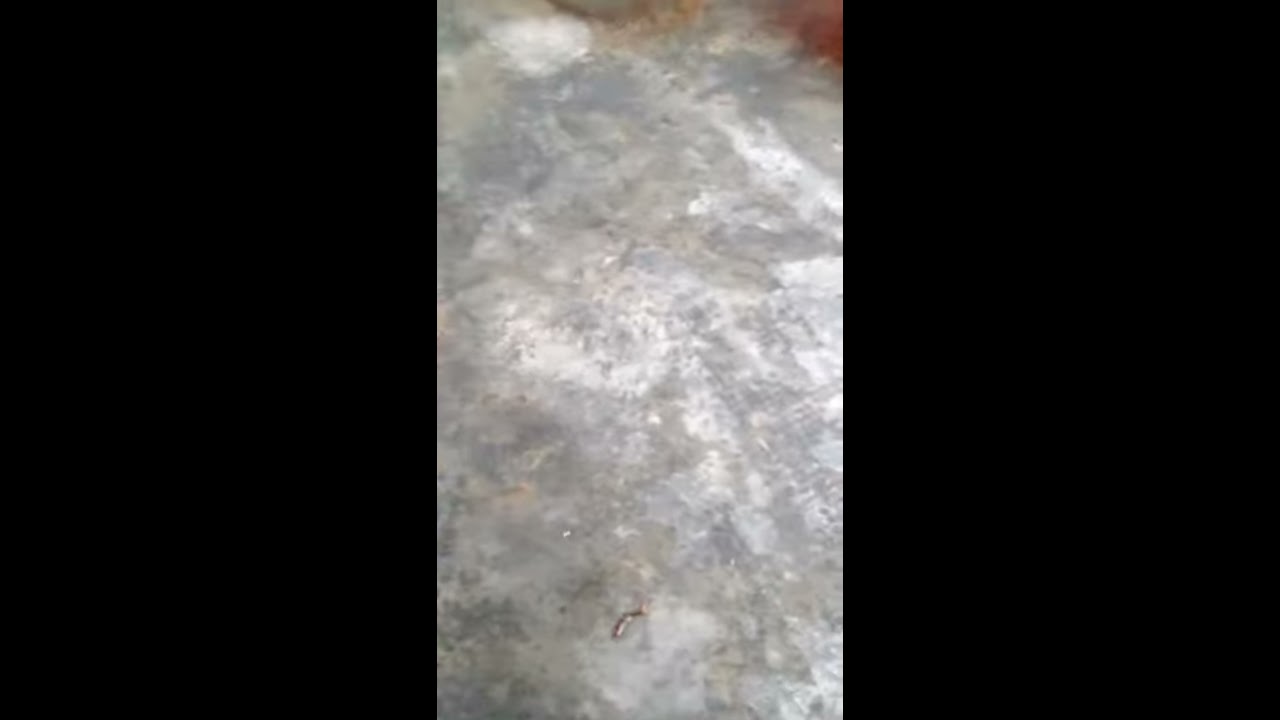This image features a predominantly black background with two black rectangles on either side, framing a central vertical panel. The middle section is a mixture of gray and white tones that resemble either a patch of concrete or possibly an icy surface. The texture is blotchy and faded, with subtle hints of silver and occasional hints of brown. Near the foreground, there's a small indistinct object, possibly a dead bug, blending with the grayish surroundings. The overall scene lacks additional elements, focusing solely on the central mysterious surface and the tiny object within it.